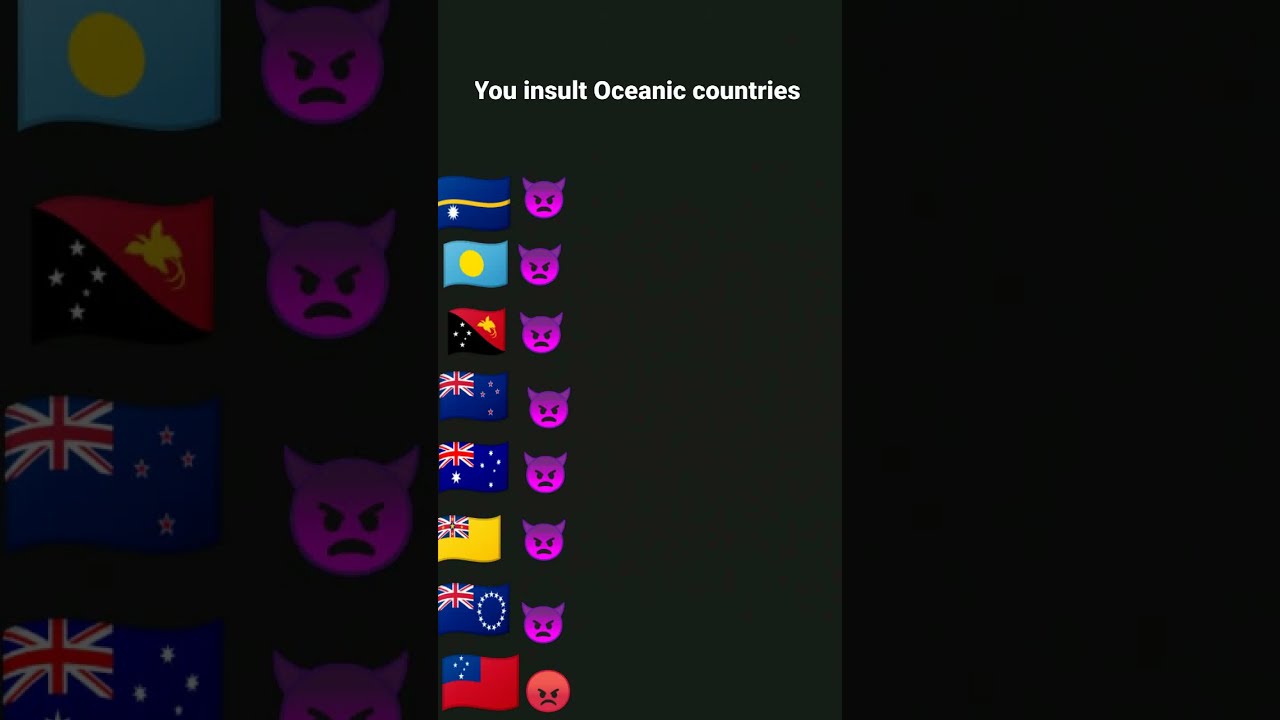This image is a tall, narrow screen grab, likely a meme or a screenshot from a video, with prominent text at the top stating "you insult oceanic countries." The central part of the image features a vertical sequence of flags, each accompanied by an angry emoji. Most of these emojis are small, purple, devil-like figures with frowning faces and horns, except for the one at the very bottom, which is a larger red emoji with an extremely angry expression. The flags, starting from the top, include:

1. A blue flag with a yellow wavy stripe horizontally across.
2. A light blue flag with a yellow circle in the middle.
3. A flag that is half black, half white at diagonals.
4. Multiple flags resembling British colonial ensigns, including one with a blue background and white stars, one fully blue, and another fully yellow with a British Union Jack in the upper left corner.

The image is bordered by a large, black rectangular box on the right, while the left side is framed by an enlarged, grayed-out portion of these flags.